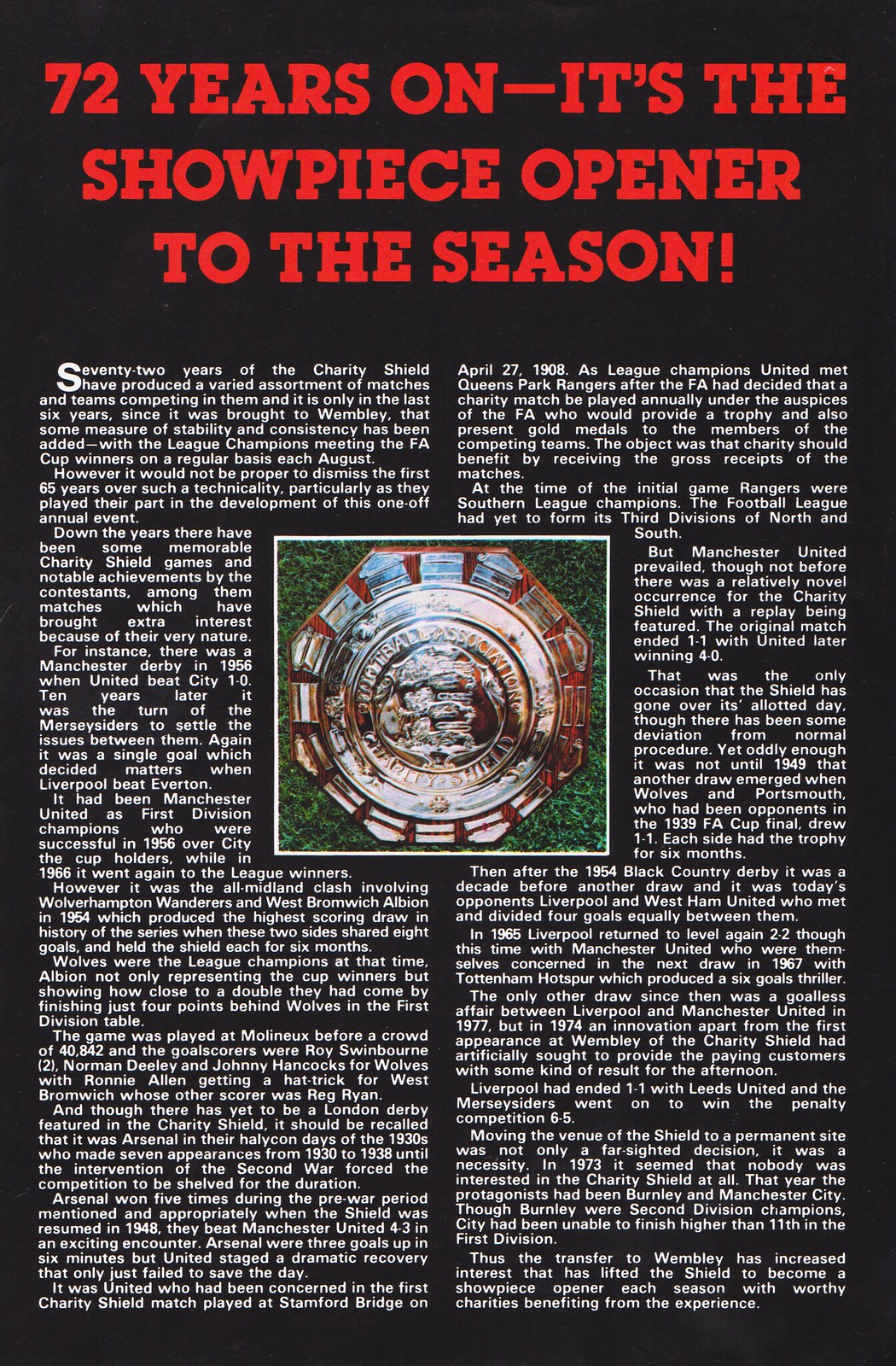The image features a large black page with an article written in white text, divided into two columns. Dominating the top of the page, bold red text reads: "72 years on, it's the showpiece opener to the season." Underneath is a detailed paragraph describing the history of the charity shield, emphasizing 72 years of diverse matches and the consistency brought about since its venue change to Wembley. Centrally placed within the article is a full-color photograph of a shield set against a green grass background, outlined in white. The shield itself is metallic and adorned with silver, red, and possibly gold elements, including an emblazoned emblem. Additionally, the text mentions "Manchester United" several times and includes a date, April 22nd, hinting at a significant event or game. The overall layout and content suggest that this page is likely taken from a game day magazine or a similar soccer-related publication.